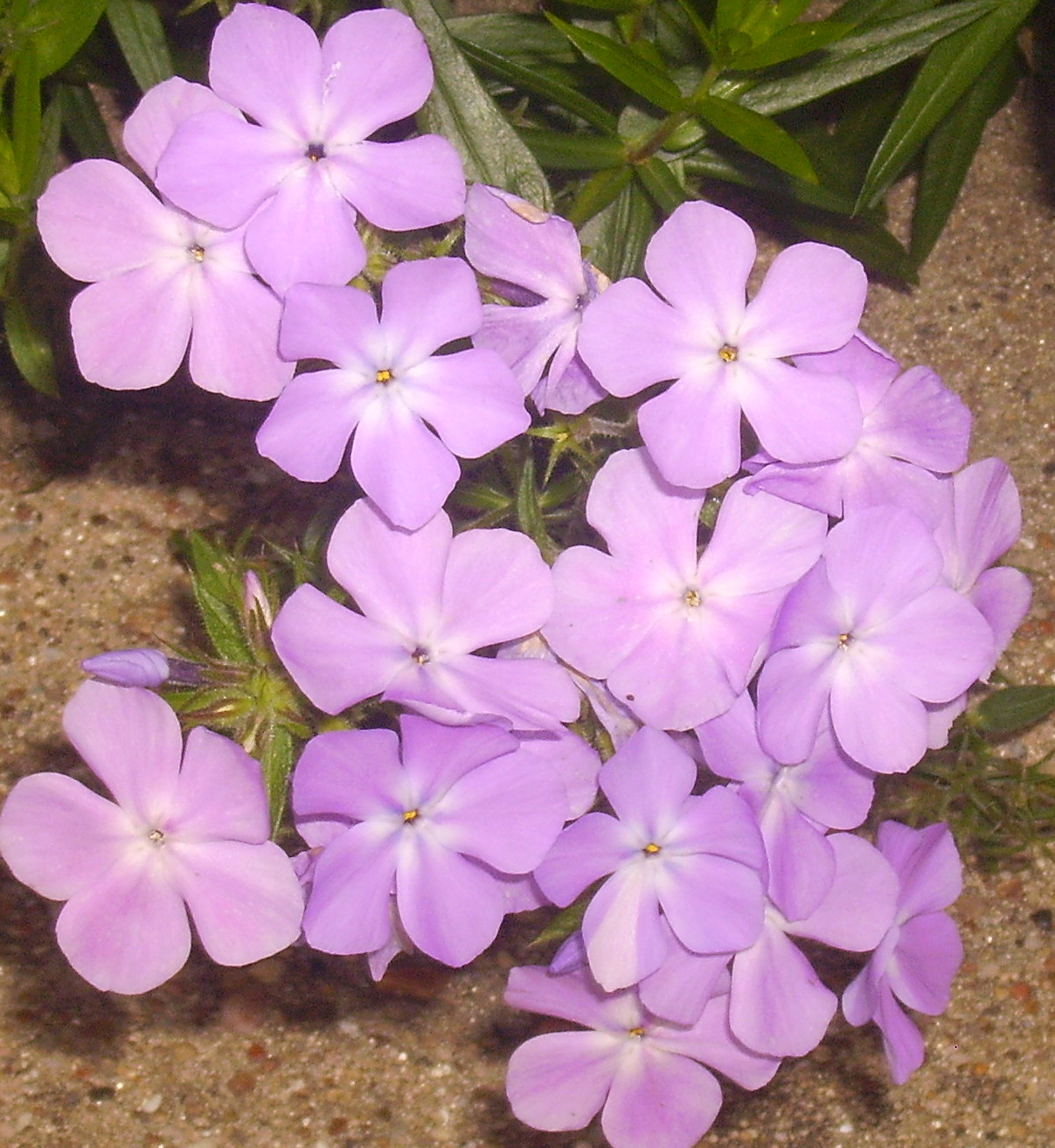This photograph showcases a vibrant cluster of purple flowers, likely Hawaiian lilies, with no people or text present. The flowers exhibit a stunning gradient, transitioning from a darker purple at the tips of their five petals to a light purple and nearly white at the center, where a yellow stamen emerges. These blossoms are nestled among lush, healthy green leaves and stems, creating a rich contrast with the flowering petals. The plant appears well-rooted in a sandy, stony substrate that might be interspersed with small, rounded rocks, suggesting a beach-like or gravelly environment. The flowers are casting faint shadows on the ground, enhancing the depth and texture of the scene.